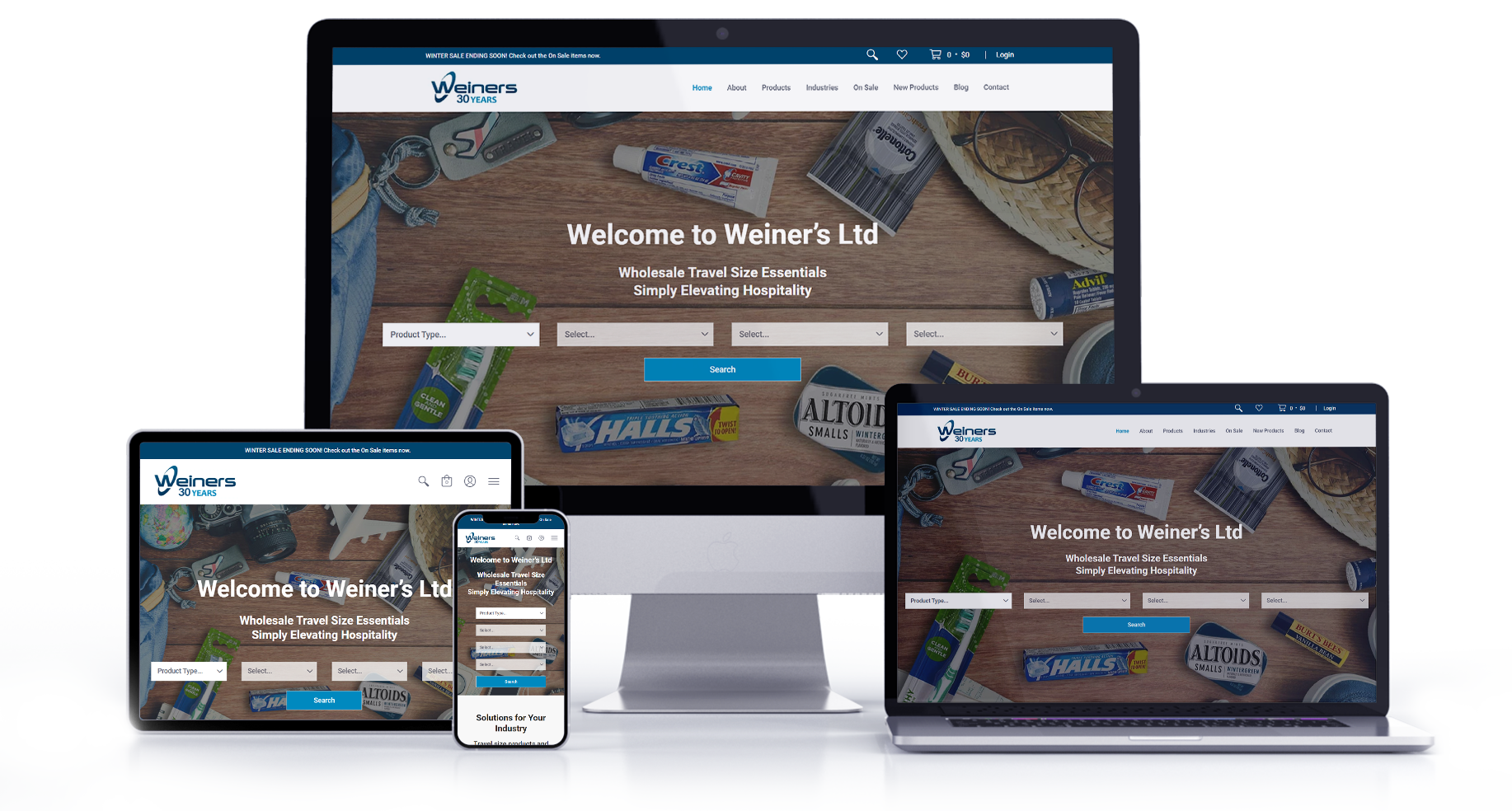A collection of advertisements for Wiener's 30th anniversary is showcased on multiple devices to illustrate the consistency and adaptability of their digital campaign. Starting from the left, a desktop computer monitor displays the ad, followed by a laptop, a tablet, and finally a smartphone on the far right. Each device exhibits the ad's user interface, highlighting how it appears across different screens.

The ad itself features a top navigation bar with options such as Home, About, and other sections relevant to Wiener's offerings. Central to the design is a visually appealing table scene set against a background that evokes the theme of travel. On the table, there is a blue travel bag adorned with a visible tag, surrounded by various travel essentials. These include Altoids mints, Crest toothpaste, Halls cough drops, and a small tube of Advil, among other items, all neatly scattered to enhance the travel aesthetic. A pair of sunglasses sits atop the brim of a straw hat, completing the travel-ready ensemble.

The ad not only highlights Wiener's long-standing reputation but also emphasizes the ease with which customers can click on and source the products depicted. This demonstration effectively shows potential customers what to expect from Wiener's digital marketing campaign across different platforms, underscoring the brand's adaptability and user-friendly approach.